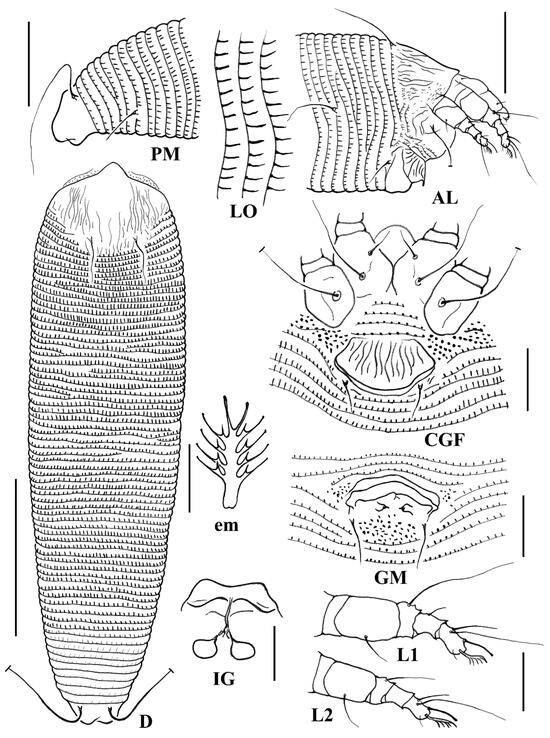This image appears to be a detailed, black-and-white pen and ink illustration from a book, depicting various anatomical parts of an insect. Across the top of the image, a series of letters such as PM, LO, AL, CGF, GM, L1, and L2 are prominently labeled, possibly representing different sections or components of the insect's body. The illustration consists of multiple detailed drawings, including a larger, oval-shaped central body part labeled PM and adjacent segments with labels like EM and IG. Some of the drawings seem to focus on the tail end of the insect, featuring detailed patterns and intricate structures. Overall, the image likely serves to inform viewers on the biological organs and functional parts of an unidentified, possibly rare or prehistoric insect, offering close-up views of various elements, including antennas, though without descriptive text to explain the significance of each part.